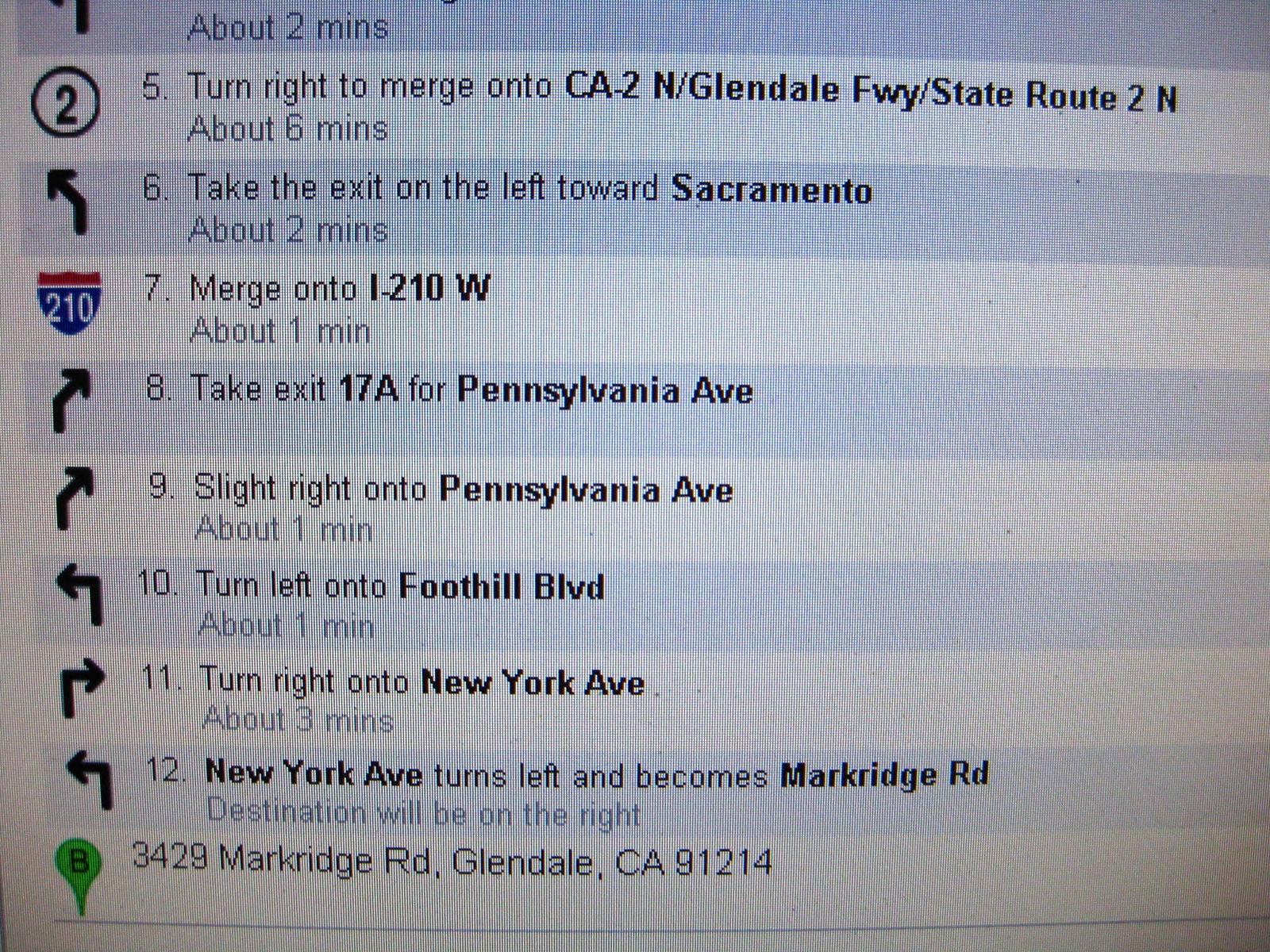In the image of a computer screen, likely taken using a camera given the visible graining, directions are displayed in a format resembling MapQuest. The directions are shaded in alternating blue and white horizontal lines, with the top portion and initial steps cut off, showing steps 5 through 12. At the top, it indicates a duration of about two minutes, and includes the distinctive feature of a number two in a circle. The final destination is 3420 Mark Ridge Road, Glendale, CA, California, 91214. Key steps involve:

1. Turning right to merge onto CA-2 North, Glendale Freeway, State Route 2N, for about six minutes.
2. Taking the exit on the left towards Sacramento.
3. Merging onto I-210 West.
4. Taking exit 17A for Pennsylvania Avenue.
5. Sliding right onto Pennsylvania Avenue.
6. Turning left onto Foothill Boulevard.
7. Turning right onto New York Avenue.
8. Noting that New York Avenue turns left and becomes Mark Ridge Road.

The destination will be on the right-hand side, and the screen features multiple arrows indicating turns, some curving to the left and others to the right, with estimated travel times for each segment.